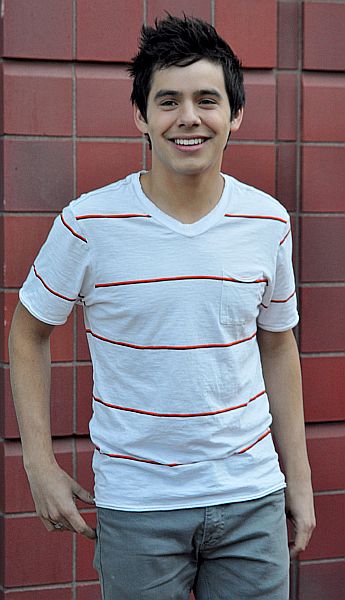The image features a young white man standing in front of a red tiled wall composed of distinct, larger-than-typical, square bricks. His short black hair is stylishly spiked up at the front, and he sports a broad smile that reveals the top row of his teeth. He wears a white short-sleeved V-neck t-shirt adorned with evenly spaced horizontal red stripes—six across the front and two on each sleeve—along with light grey jeans. The man is centered in the picture, with his body facing forward slightly towards the viewer’s right. His right elbow is slightly bent with his hand near his pocket, while his left arm hangs straight down. The wall forms a clean backdrop, emphasizing the man’s relaxed yet engaging pose. The image is cropped to show him from the top of his head to just above his knees.